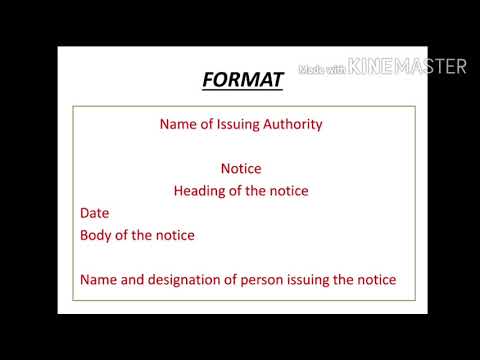The image is predominantly a white slide framed by a thick black border. At the top of the slide, in bold, italicized, uppercase black letters, the word "FORMAT" is prominently displayed and underlined. Below this heading, there is a rectangular section containing red text which outlines a template for an official notice. The red text reads: "Name of issuing authority, Notice, Heading of the notice, Date, Body of the notice, Name and designation of person issuing the notice." This text appears to serve as a guide for drafting formal documentation. Additionally, at the upper right corner of the image, there is a watermark stating "MADE WITH KINEMASTER" in all uppercase letters, indicating that the video editing software KineMaster was used to create this slide. The entire image is bordered by a thick black line, adding to its structured and organized appearance.